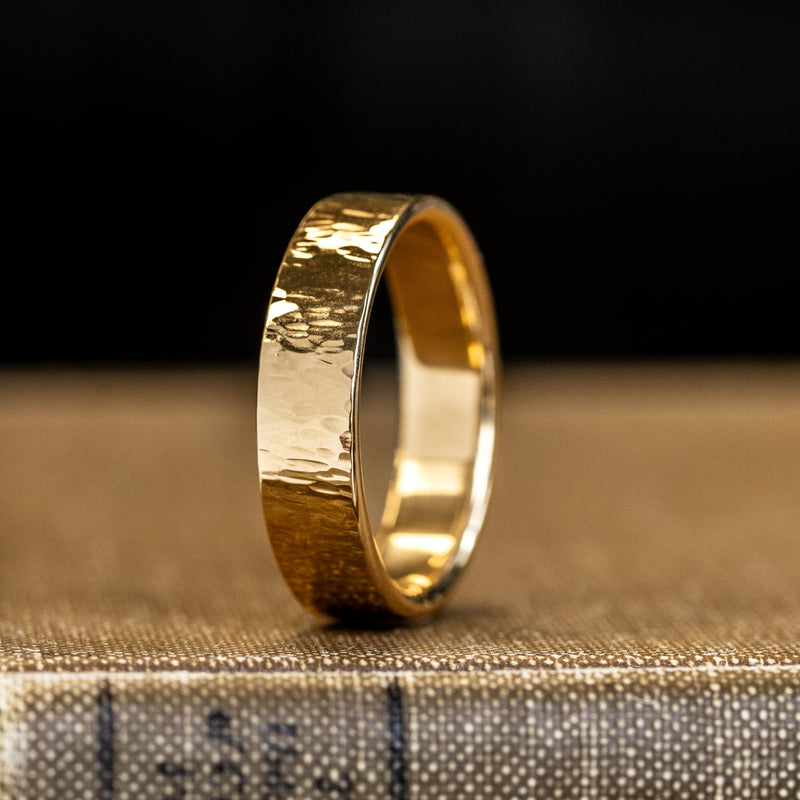This image is a very close-up, highly detailed photograph of a gold ring, standing on its edge. The ring appears to have a hammered or etched pattern, with horizontal ridges and slight rivets around its band, giving it an older, textured appearance. The gold surface is highly reflective, capturing and reflecting the light in the room, with some reflections appearing almost silver. The ring's interior and right side are especially shiny.

The gold band is positioned on the cover of a brown, hardbound book, which features a speckled pattern with white pitted marks. The spine of the book is darker brown with two vertical black lines and some black cursive text, although the inscription remains indecipherable due to the extreme zoom and angle of the shot. The book’s surface is in sharp focus in the foreground, while the background, which is plain black and slightly blurry, fades into softness, ensuring the golden ring stands out as the primary subject of the image.